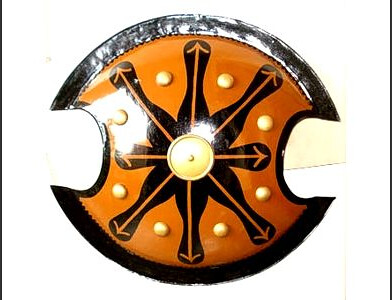The image features a circular object that resembles either a modern interpretation of an antique Asian martial arts weapon or a decorative adornment. The circular shape is interrupted by two C-shaped cutouts on opposite sides, making it not a complete circle. The outer rim is black, while the interior displays an orangish-brown hue, giving a glossy and shiny appearance. The center of the circle is highlighted by a gold button-like feature with a prominent dot. Radiating from this central gold element are eight black, elongated shapes, each directed outward like spokes or compass points, with orange arrows extending from them. Between these shapes, gold studs are strategically placed, adding to the ornate design. The background is plain white, suggesting the image may have been digitally altered to remove any surrounding context, making the object stand out more prominently.